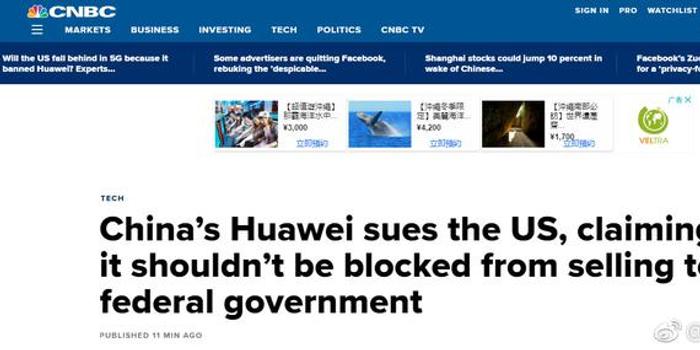Cropped Screenshot of the CNBC Website

The image depicts a cropped screenshot of the CNBC website, showcasing only the top left quarter of the homepage. The top bar is characterized by a blue background, displaying various sections including "Markets," "Business," "Investing," "Tech," "Politics," "CNBC," and "TV." On the right side of the top bar, there are buttons labeled "Sign In," "Pro," and "Watchlist."

The visible portion of the page prominently features a key headline under the "Tech" section: "China's Huawei says the US should not block it from selling to the federal government," which was published 11 minutes ago. Additional headlines are displayed in a marquee-like format near the top of the screen, including "Will the US fall behind in 5G because it banned Huawei?" "Some advertisers are quitting Facebook," and "Shanghai stocks could jump 10%," with the last headline about Facebook being partially cut off.

A banner ad with Chinese or Asian characters is also visible on the page. The predominant color scheme of the webpage is white, and it clearly serves as a platform for finance-related news, including stocks and market updates. Several images are present, including one depicting a whale breaching, although the accompanying text is not discernible.